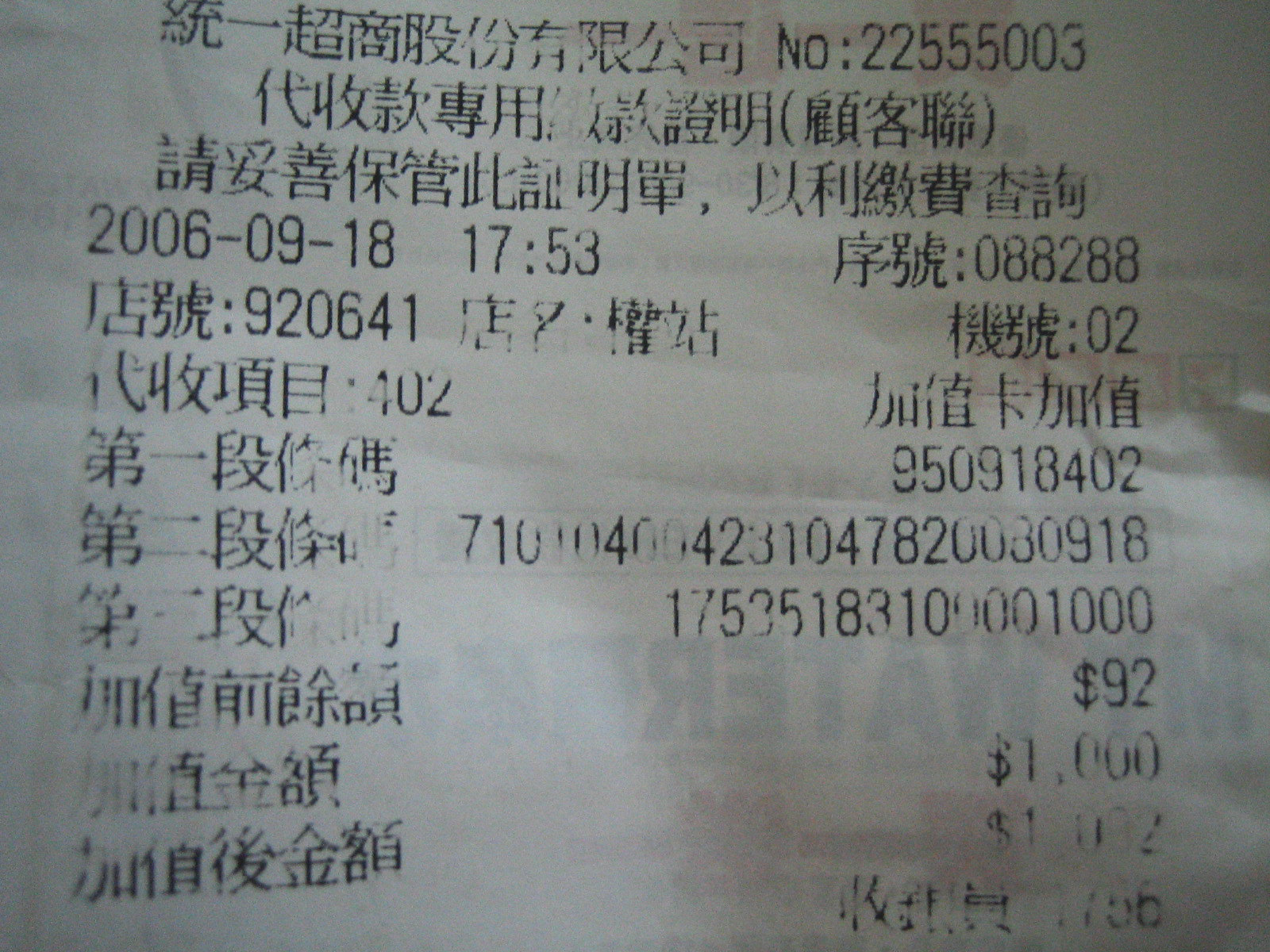This image, which is wider than it is tall, features a mix of Chinese characters and Western-style numerals, strongly suggesting that it is a receipt or a bill of sale. Dominating the top portion is a lengthy string of Chinese characters. In the top-right corner, there's a notable detail in Western lettering: "N-O:" followed by the number "22555003."

Throughout the document, a combination of Chinese characters and numerical digits is evident. Noteworthy entries include the date "2006-09-18" and the time stamp "17.53," indicating 5:53 PM on September 18, 2006. On the right-hand side of the image, there are financial figures listed as "$92" and "$1,000," reinforcing the notion that this document is likely a receipt detailing multiple transactions.

Overall, the precise arrangement of dates, times, and monetary values, interspersed with Chinese text, provides a detailed snapshot of a financial exchange, capturing the recorded details meticulously.